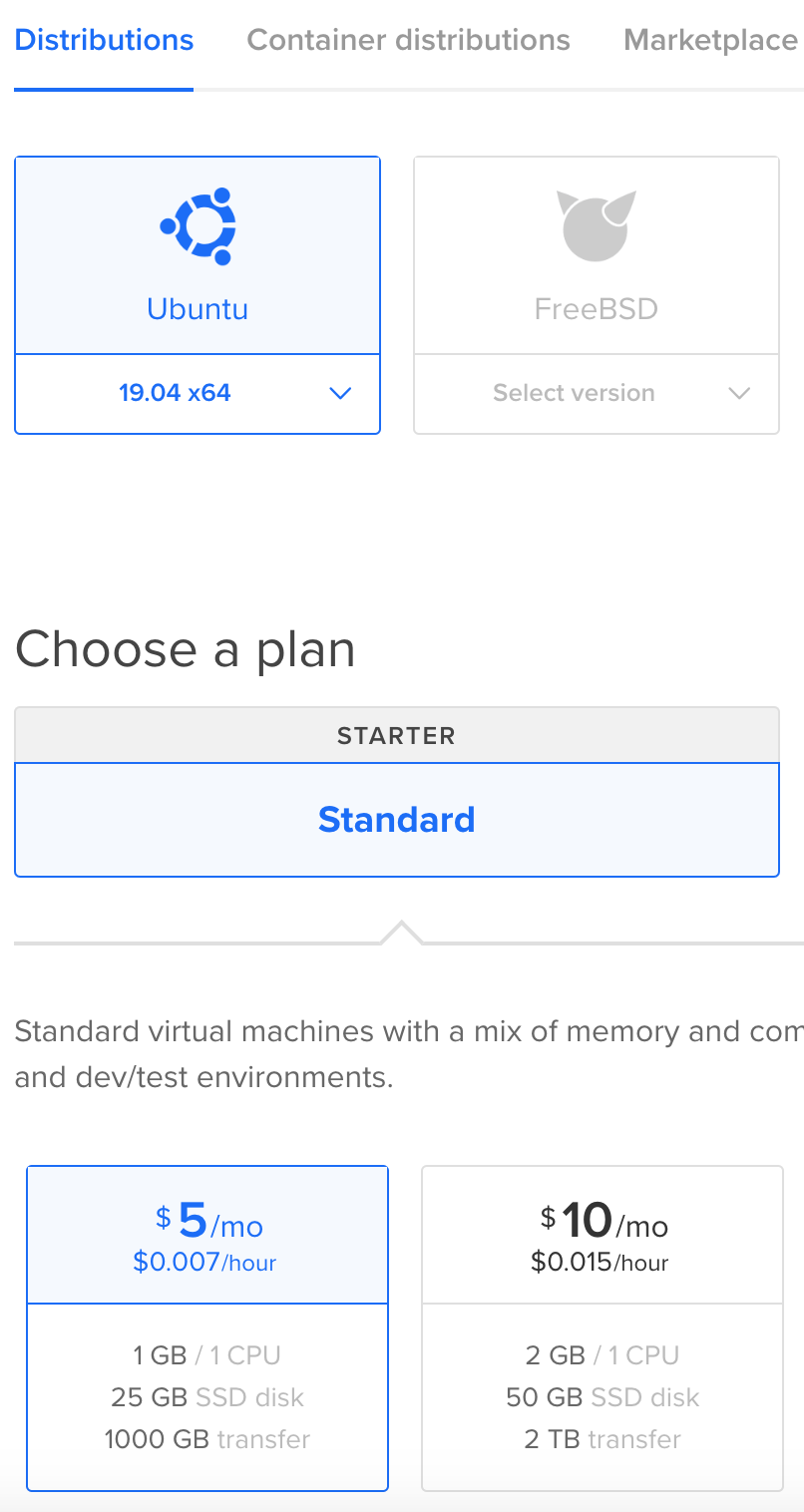This is a detailed descriptive caption for the image provided:

The image is a screenshot of a smartphone displaying a plan selection page. The background is predominantly white. At the top of the screenshot, there is a header with three labels arranged horizontally: "Distributions," "Container Distributions," and "Marketplace." The label "Distributions" is highlighted in blue with a blue underline, indicating it is the currently selected tab.

Below the header, there are two selection boxes. The first box, highlighted in blue, features a circular logo with three dots on the perimeter, labeled "Ubuntu." Beneath this is a dropdown menu currently showing "19.04 X64." The second box, in light gray, is labeled "FreeBSD" and contains a scroll bar for selecting a version, indicating it is not selected.

Centered in the image is a prominent header that reads "Choose a Plan." Under this header is a light gray box with the label "Starter." Adjacent to this is a blue button reading "Standards." Below this section, separated by a line, is additional text that begins with "Standard Virtual Machines with a mix of" but is partially cut off on the right side. The readable portion continues with "dev/test environments."

Beneath this section are two plan options. The first plan, highlighted in blue, costs $5 per month and includes specifications of 1 GB of memory, 25 GB of SSD disk space, and 1,000 GB of transfer. The second plan, in an unselected gray box, costs $10 per month and includes 2 GB of memory, one CPU, 50 GB of SSD disk space, and 2 TB of transfer.

Every element is accurately aligned with no visible borders around the image, emphasizing the clean and organized layout of the page.